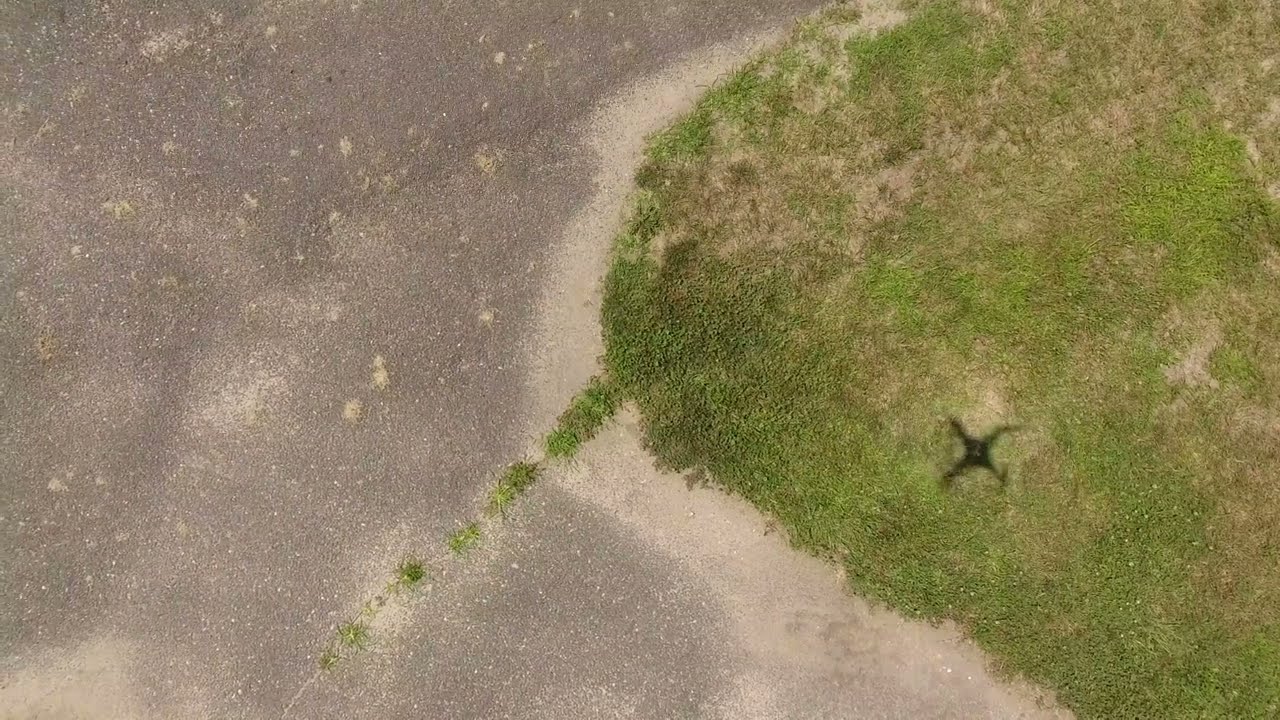The image captures a close-up view of a yard taken from above, likely from a drone. The scene features a curved patch of grass, predominately lime green but mottled with patches of brown dirt, hinting at a mix of healthy and dead grass. This grassy area is juxtaposed against a light gray concrete pavement situated on the left side, where tufts of grass emerge through a crack. A prominent shadow, resembling a drone or potentially a ninja star, casts over the grass, suggesting that the photo may have been taken from a drone. The overall composition is simple, free of people and text, highlighting the contrasting textures of the concrete and grass with a sandy outline subtly delineating the two surfaces.